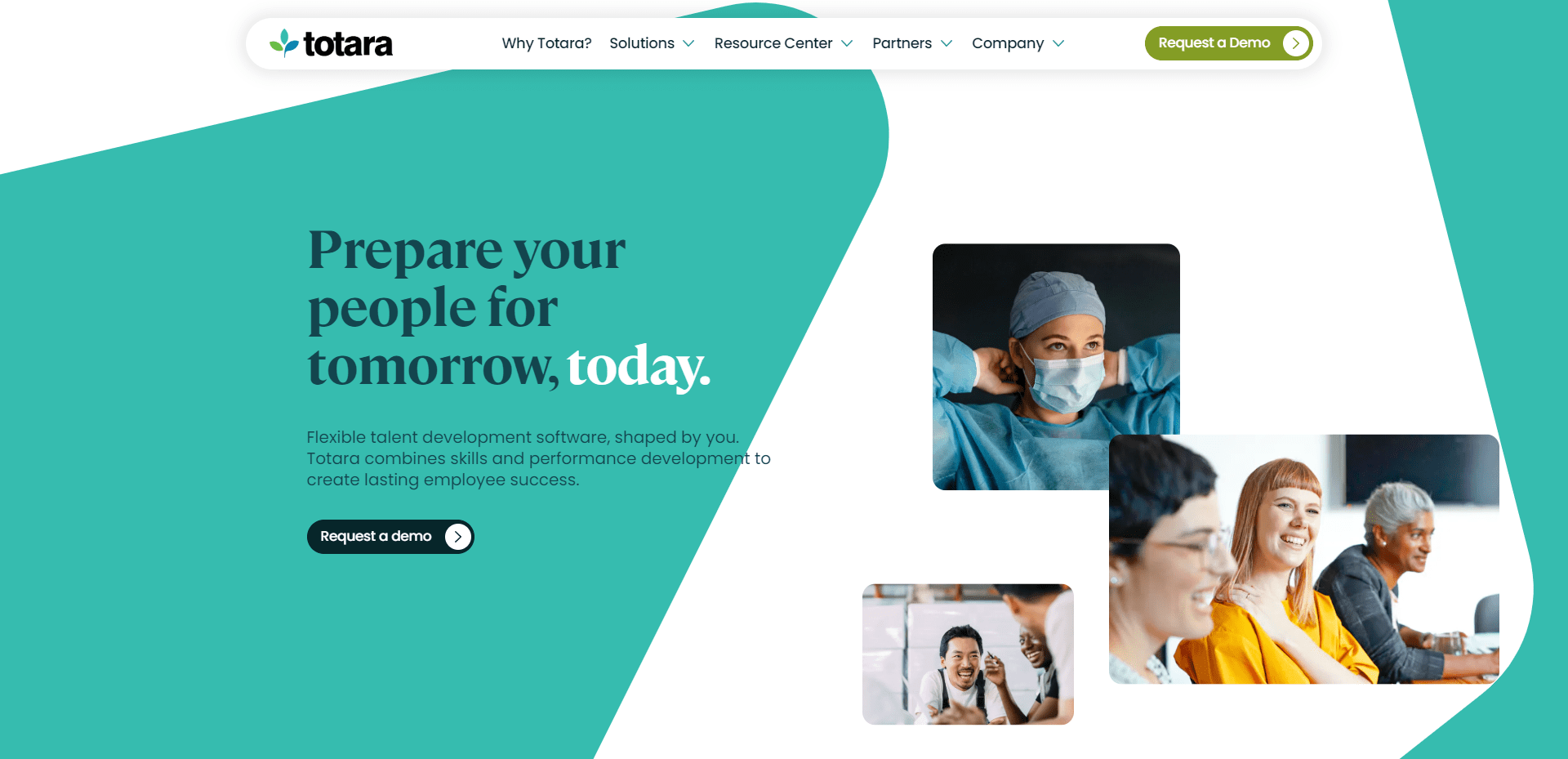The image depicts a sleek, professional webpage from Totara, characterized by a long rectangular layout. At the top, there is an elongated oval menu bar, centrally featuring the Totara logo. This menu bar includes several items: 

- "Why Totara" 
- "Solutions" (with a drop-down arrow)
- "Resource Center" (with a drop-down arrow)
- "Partners" (with a drop-down arrow)
- "Company" (with a drop-down arrow)

To the right of these options, there is a prominent green button labeled "Request a Demo" in white font, accompanied by a circular icon with an arrow pointing to the right.

The background of the webpage is an engaging aqua blue, adorned with simple, clean white designs that enhance its modern look. Toward the left side of the page, there is a compelling white headline stating "Prepare your people for tomorrow. Power today." directly below it, in a dark blue font, is the line "Prepare your people for tomorrow."

Under this headline, a body of text elaborates on the stated theme. Just beneath this text, there's another "Request a Demo" button similar to the one in the top menu. Additionally, the design features three images of people from various backgrounds, indicating diversity and inclusion.